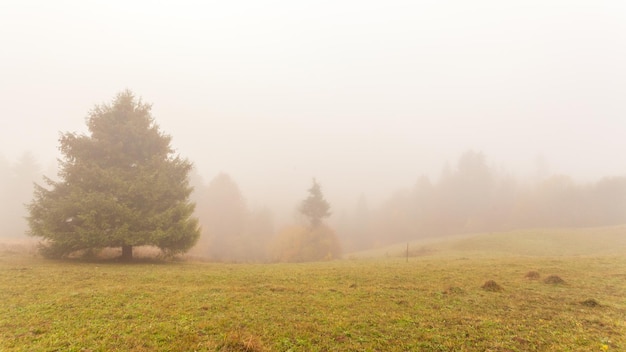This photograph captures a fog-enshrouded landscape, characterized by a low, rolling field that gently slopes downward. The foreground reveals a mix of short, yellowish-brown grass interspersed with small mounds, possibly molehills or clumps of dead grass. Dominating the left side of the image is a large, conical pine tree, approximately 30 feet tall, partially obscured by the dense fog that blankets the area. The fog is so thick that visibility extends no more than 200 yards, rendering the sky invisible and the colors muted. In the background, a line of trees fades into the fog, becoming mere shadowy silhouettes against the increasingly opaque white and gray mist. This creates a haunting yet serene atmosphere where details blur and the horizon is lost to a thick, enveloping shroud of fog.